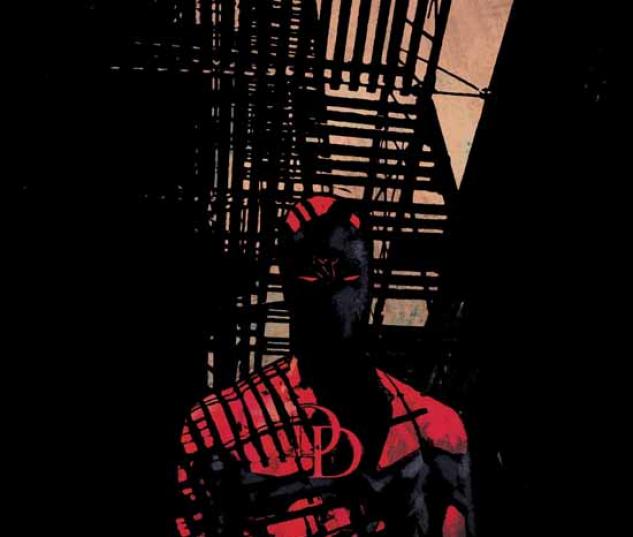This photograph, likely an artistic rendition from a comic book, depicts the iconic character Daredevil, instantly recognizable by the "DD" emblazoned on his tight red costume. The image is shrouded in darkness, with Daredevil standing centrally beneath what appears to be a metal fire escape or scaffolding, indicative of a gritty urban environment, possibly a New York City alley. The sparse lighting filters through the black grid of the steps above, casting reflective stripes and a harsh shadow over Daredevil, only accentuating his menacing silhouette. His face is obscured by a black mask, with piercing red slit eyes glaring from the darkness. The prominent black stripe across his chest further adds to his imposing figure, blending with the shadows and the reflective grid patterns.